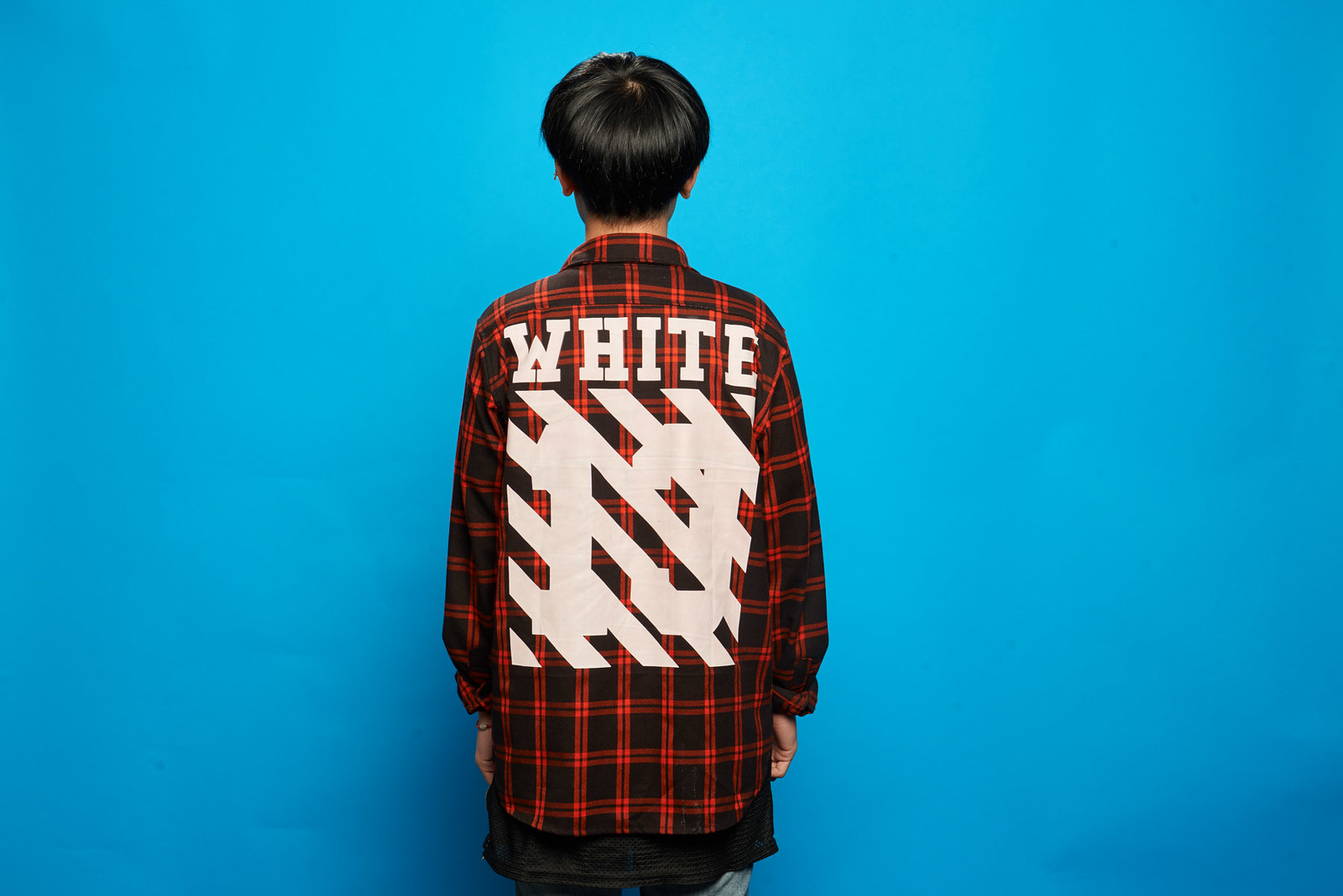In this image, we're observing the back of a person facing a predominantly sky-blue background, which becomes slightly darker towards the bottom right corner. The subject, oriented in a landscape frame, has short black hair, neatly trimmed around the neck and just brushing the top of the ears. They wear a long, dark red and black plaid flannel shirt. Across the shoulders of the shirt, in bold uppercase white letters, is the name "WHITE". Beneath this, where an athlete's number might typically appear, is the number "13", struck through with white diagonal lines running from the bottom left to the top right. The person’s hands rest by their sides, and you can glimpse a black shirt layered underneath the plaid flannel. The individual appears to be wearing gray pants, completing the outfit.